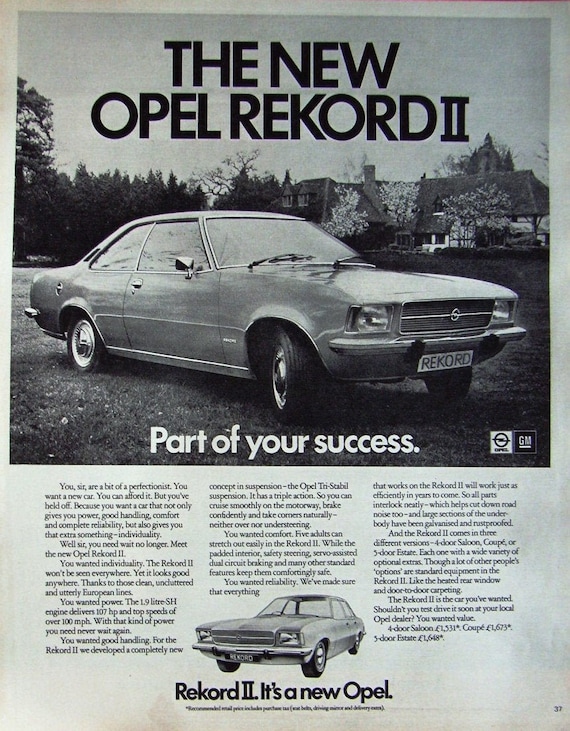This black and white advertisement from the 1960s promotes the new Opel Rekord 2 by General Motors. The vertically rectangular image is divided into two main sections. The top two-thirds feature a photograph of the stylish, two-door Opel Rekord 2 parked on a grassy field in front of a large house with trees in the background. Despite the monochrome palette making the exact color of the car indiscernible, its sleek design is clearly the focal point. Above the car, bold black text reads "The New Opel Rekord 2", emphasizing the model's novelty. In the bottom third of the ad, several paragraphs of text extol the car's attributes, although the finer details are difficult to read. Centered at the bottom, the slogan "Part of your Success" in white reinforces the branding message, accompanied by the General Motors logo. The overall presentation suggests sophistication and reliability, appealing to discerning customers of the era.